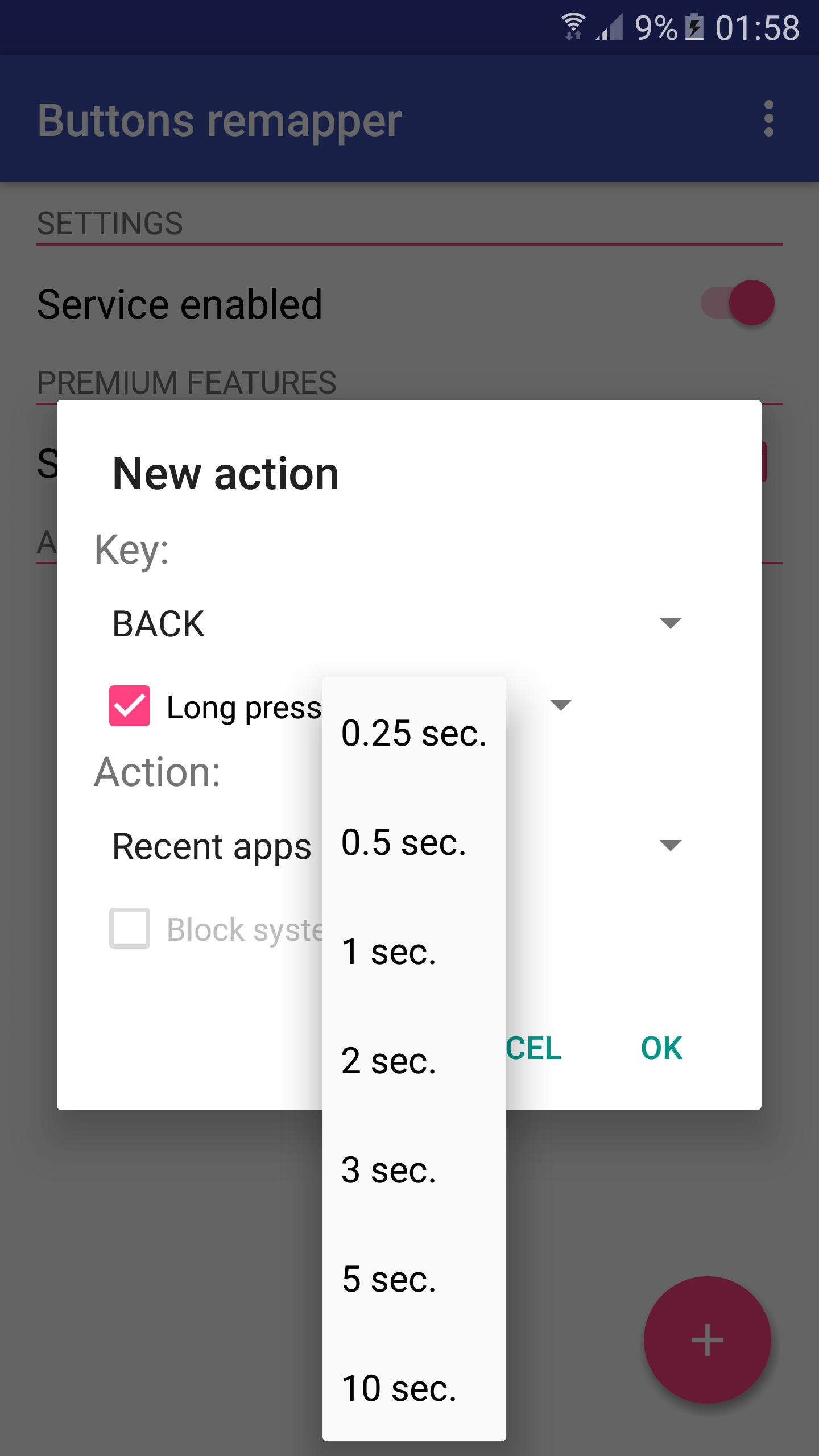The image is a screenshot taken from a phone, primarily showcasing a user interface with various settings and options. The background is slightly grayed out, with the top portion featuring a dark blue bar. On the right-hand side of the status bar, there are icons indicating full Wi-Fi connectivity, two bars of cell service, a low battery at 9%, and a charging icon. The time displayed is 01:58 AM.

Beneath the blue bar, the background shifts to a lighter blue, and on the left side, the text "Blue Remapper" appears in white, accompanied by a three-dot menu icon. The main interface has a white background with a gray line separating different sections. In darker font, the text "Service Enabled" is shown with a toggle switch to its right, which is currently enabled. Below this, in gray text, it states "Premium Features."

A white pop-up box is present with the heading "New Action" in black text. Within this box, there is a gray label "Key" followed by a dropdown menu where "Back" is selected. Additionally, there is a checkbox next to the option "Long Press." Another smaller pop-up window contains various time intervals in black text: 0.05s, 0.5s, 1s, 2s, 3s, 5s, and 10s. 

Back on the main interface, the word "Action" is shown in gray, followed by a dropdown labeled "Receipt Apps." Partially visible buttons towards the bottom include a square with "SYS" and possibly "System," and another button with "CEL" which is partially obstructed, likely indicating "Cancel." To the right of these, there is a clearly visible "OK" button.

In the bottom right corner of the grayed-out background area, a red circle with a white plus sign is prominently displayed, suggesting an option to add more actions or settings.